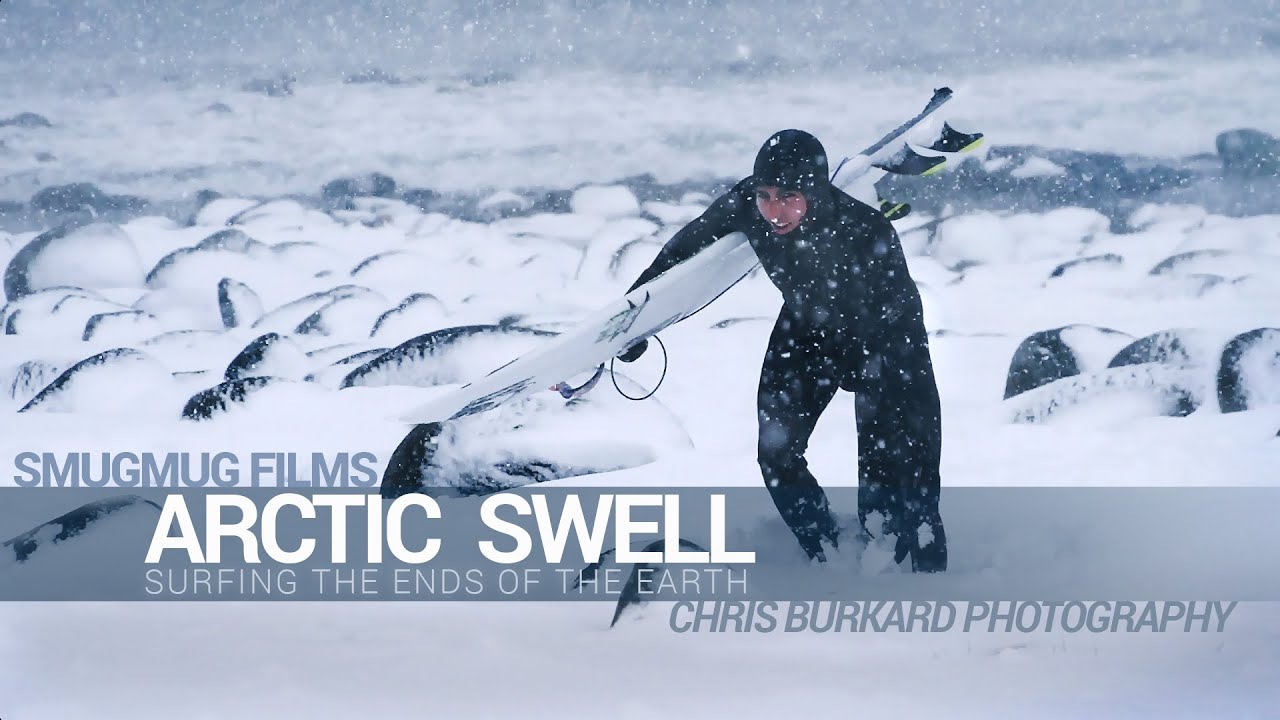The image is a promotional photograph for "Arctic Swell: Surfing the Ends of the Earth," produced by Smug Mug Films with photography by Chris Burkhart. In a snowy, blizzard-like setting, a man is depicted wearing an all-black wetsuit with a matching helmet and gloves, suggesting he's prepared for extreme cold conditions. He holds a large white surfboard. The ground and background are blanketed with snow, and various rock formations, partly covered in snow, are visible. Scattered in the distance are dark, indistinct shapes, possibly dead penguins, adding to the harsh and remote feel of the scene. The text "Arctic Swell: Surfing the Ends of the Earth" is prominently displayed in a darkened box that spans the width of the image, enhancing the dramatic and adventurous tone of the portrayal.